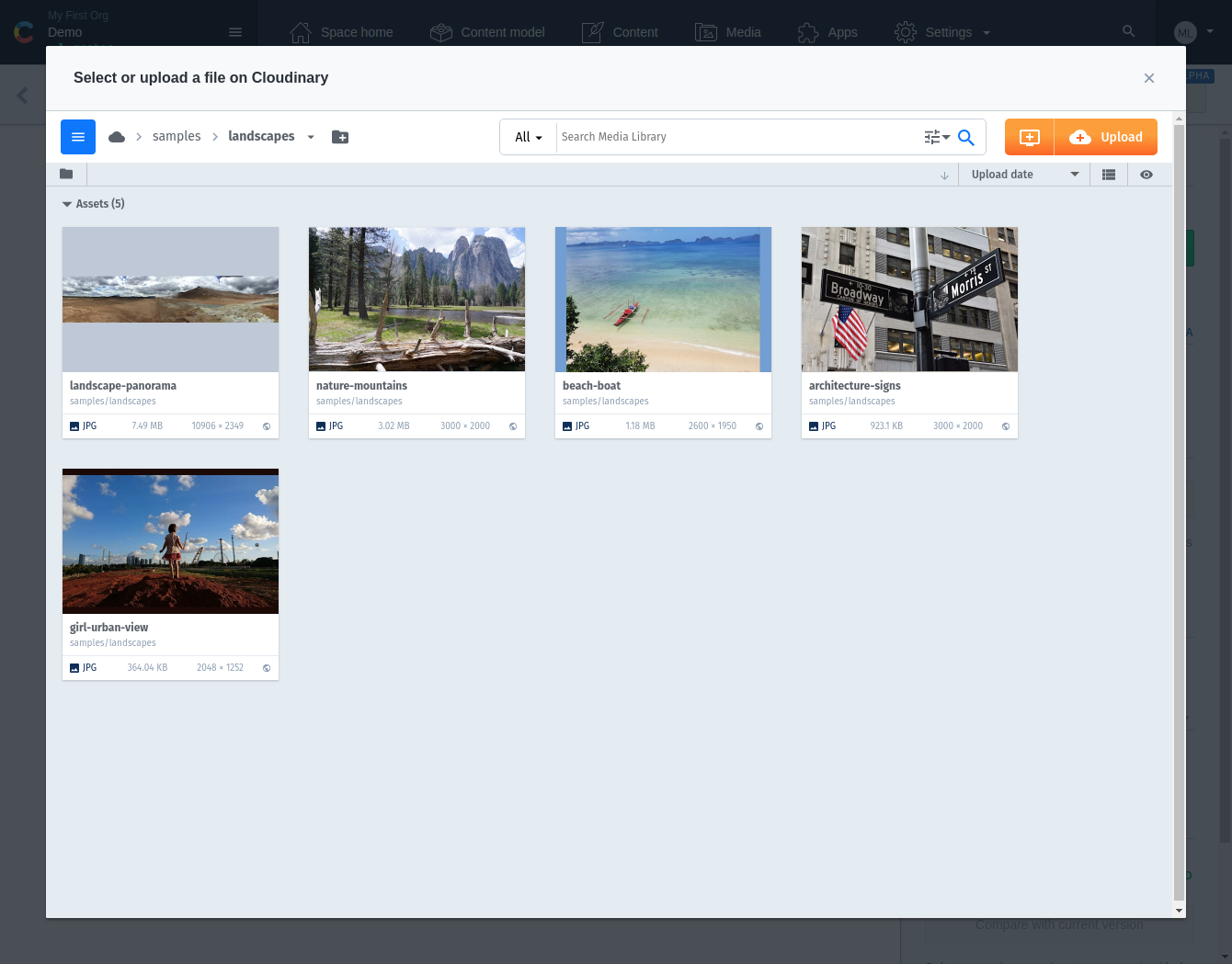The image displays a large pop-up window that nearly covers the entire webpage, making it difficult to see much of the background, which is a subtle gray. The pop-up itself features a very light bluish-gray hue.

At the top of the pop-up, a black bar displays the text "Select or upload a file from Clowndon." A thin gray line separates this section from the rest. Below, there is a blue square containing three white horizontal lines, positioned next to a gray cloud icon. The word "Samples" follows in gray, alongside the term "Landscapes."

To the left, a white search box features the word "All" in black text. Adjacent to this, in gray, it reads "Social Media Library," and a blue magnifying glass icon is present for search functionality. Below this, an orange rectangle showcases a white cloud and an orange plus sign with the word "Upload" written in white.

The pop-up’s background transitions to a deeper gray, displaying the word "All" followed by "(5)" in parentheses, indicating the number of images present.

The five images are laid out as follows:
1. The first image depicts brown mountains against a sky with white clouds. Beneath this image, the text "landscape-panorama" is written in gray.
2. The second image shows a scene with doors, water, and mountains, labeled "nature-mountains" in gray text.
3. The third image captures a beach setting with sand, water, trees, and a red canoe. It is titled "beach-boat" in gray.
4. The fourth image includes an American flag and street signs reading "Broadway" and "Morris." The label "architecture-signs" appears underneath in gray.
5. The final image features a girl in a red field with the caption "girl-urban view" in gray text.